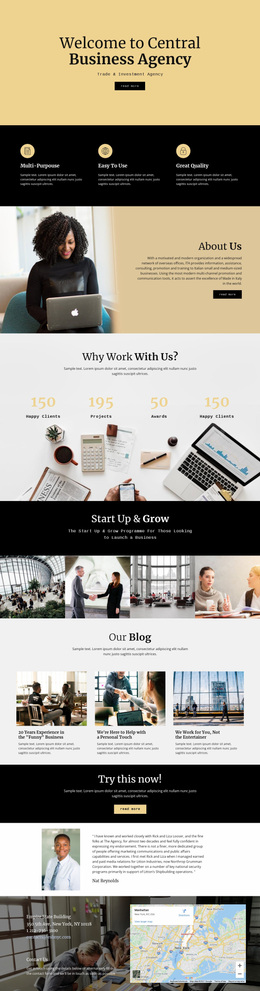This image depicts the homepage of a business agency's website, characterized by a stretched and vertically compressed layout that makes the text difficult to read due to its small size. The color scheme alternates between goldish-yellow, black, and white in a repeating pattern. 

At the top of the page, the header reads "Welcome to Central Business Agency," followed by an indistinct button. Below this header is a black banner showcasing different features with legible phrases such as "Great Quality" and "Easy to Use." 

Further down, there's an image of a woman using an Apple MacBook next to an "About Us" section. Following this, a "Why Work With Us" segment appears, listing persuasive statistics or reasons.

As the page continues to unfold, sections labeled "Start Up and Grow," "Our Blog," and "Try This Now" are visibly arranged. Towards the bottom, there is a map, adding a geographic element to the website's comprehensive and detailed layout.